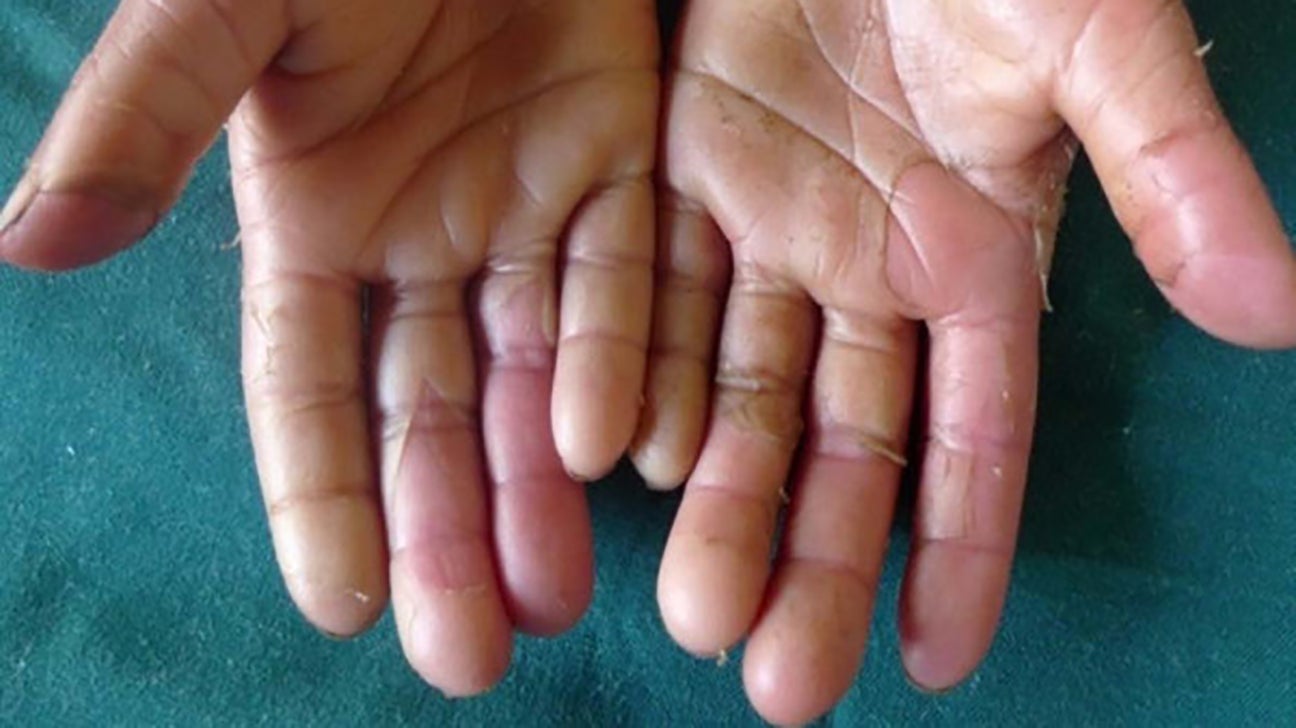This is a detailed photograph capturing the damaged hands of a person, likely a white male, who appears to have endured significant wear and tear, possibly from using tools like a shovel or an axe. The hands are held out with the palms facing up, and their thumbs positioned toward the outside of the image. While all ten fingers are visible, they are marked by severe damage: the skin is cracked, peeling, and red blisters are prominent, especially on the middle fingers and pinky fingers. The skin exhibits two distinct shades; there are areas where the skin is brown and scaly, and other regions where it’s peeled away, revealing raw, red skin underneath. The nails are reasonably well-kept, though they contain dirt and look somewhat grimy with dirt caked under them. Additionally, flakes of dead skin are scattered both on the hands and on the seafoam green or aqua blue cloth that lies beneath them. The overall state of the hands indicates extensive use and damage, with pieces of hanging skin highlighting the severity of the wear.